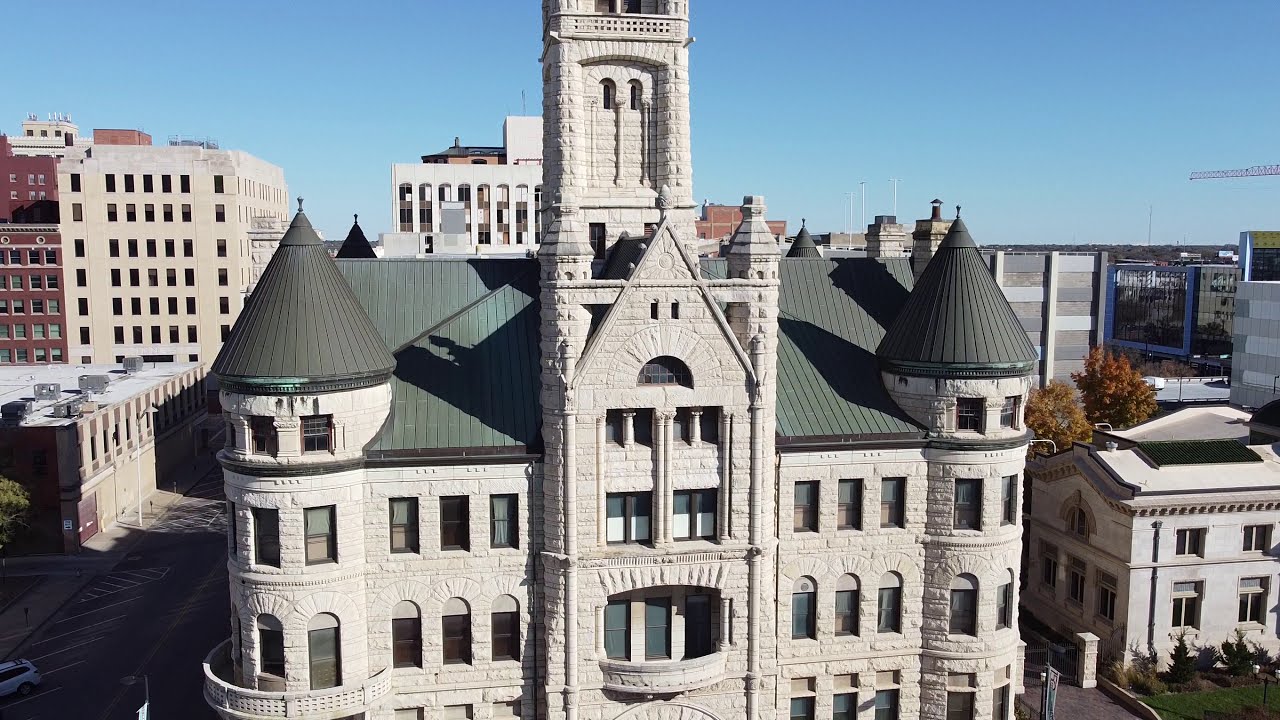In this outdoor photograph taken from high above, possibly via a drone, the focus is on a large, historic building set against a clear blue sky with minimal cloud coverage. The building, centrally featured, appears to be constructed from stone and brick, evoking an older architectural style reminiscent of a university or a church. It is several stories tall, though the street level is not visible in the image. Notably, the building has two prominent rounded turrets on either side, each capped with an upswept, cone-shaped roof that has weathered to a dark green copper patina. These turrets, which add a castle-like appearance, frame the structure's central tower, which rises straight up from the roof but extends beyond the photograph's upper boundary. Scattered square windows punctuate the walls, adding to the building’s historical aesthetic. On the far right edge of the frame, a red crane indicates ongoing construction nearby within this well-developed urban environment. Surrounding the building are other tall, multi-story structures, likely residential and office buildings, contributing to a dense cityscape.